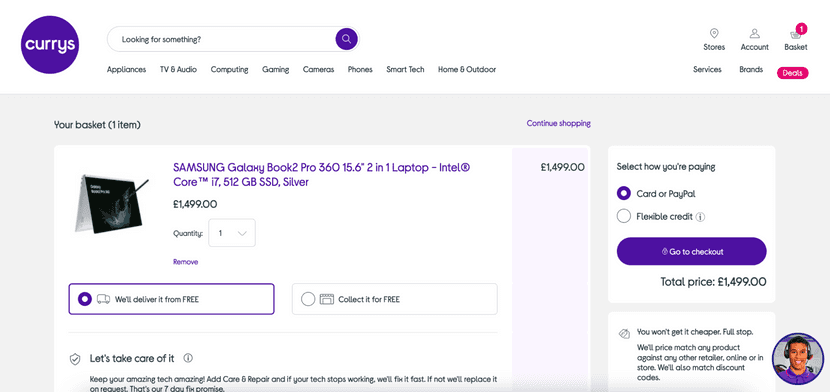The image is a horizontally rectangular screenshot showcasing the upper section of a website's item listing page. On the top left corner, there's a purple circle with the "Curry's" logo in white, indicating the website's domain. The page is currently displaying a shopping basket containing one item: a Samsung Galaxy Book 2 Pro 360, a 15.6-inch 2-in-1 laptop featuring an Intel Core i7 processor, 512GB SSD storage, in a sleek silver color, priced at £1,499. The item quantity is listed as 1, with an option below to remove the item from the basket.

Directly beneath this, there are two horizontal tabs offering delivery options. The left tab, labeled "We'll deliver it for free," is the selected option. The adjacent right tab reads "Collect it for free," providing an alternative pickup option.

On the right-hand side of the page, there’s a section prompting the user to select their payment method. The choices available are "Card or PayPal" and "Flexible Credit," with "Card or PayPal" being the currently selected option. Directly below this is a prominent "Go to Checkout" button, ready to proceed with the purchase.